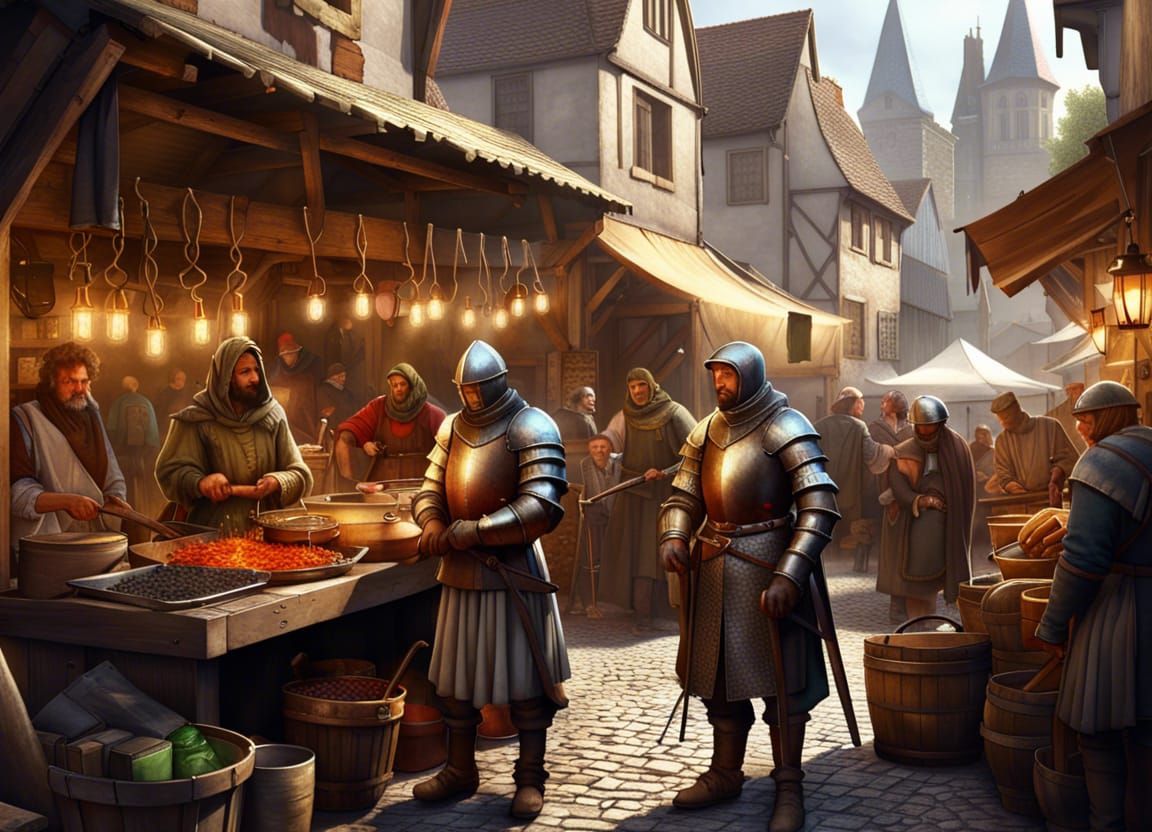This vibrant, AI-generated illustration depicts a medieval-style market bustling with activity within a narrow cobblestone alleyway. The scene is set against a backdrop of tan buildings with brown trim and roofs, and a light blue sky. In the distance, two tan towers rise above the structures. In the foreground, on the left-hand side, a food stall operated by two men catches the eye. One man, dressed in a green headscarf and long-sleeve outfit, stands beside another wearing a white long-sleeve outfit with a brown sash. They are preparing food in large pots, one orange-colored and one smaller blue pot, on thick wooden tables adorned with silver trays and wooden buckets brimming with produce. 

Two armored knights, complete with metal helmets, gloves, boots, and swords at their hips, stride through the heart of the market. These knights, possibly city guards, add to the medieval ambiance. Scattered throughout are commoners engaging with various vendors. On the right, more stalls display wooden buckets and barrels filled with bread and fresh produce. The market is lively with people and goods, creating an atmosphere that transports viewers back to an olden time village teeming with commerce and community.